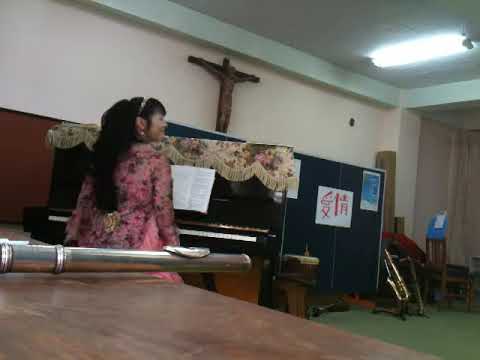In a smaller square image set in what resembles a church, an Asian woman is casually leaned against a marble-like brown table on the left side, almost leaning while smiling towards the camera. Her long, fluffy black hair is adorned with a headband and earrings, and she wears a pink floral dress that reaches mid-calf. The room is a bit cluttered, with various items such as chairs, cupboards, and musical instruments, suggesting it might be a multi-purpose or music practice room. In the immediate foreground, a shiny silver rod rests on the marbled table. A few feet in front of her, a black upright piano stands, topped with an ornate tasseled runner blanket and open sheet music, indicating she may have been playing. The floor is green tile, adding a distinct contrast to the setting. In the background, a prominent wooden cross with Jesus hanging from it is centered on a white wall, completing the church-like ambiance. There’s also a visible saxophone and some Asian writing on banners near a dark corner, suggesting the room might be in a church basement or similar area.